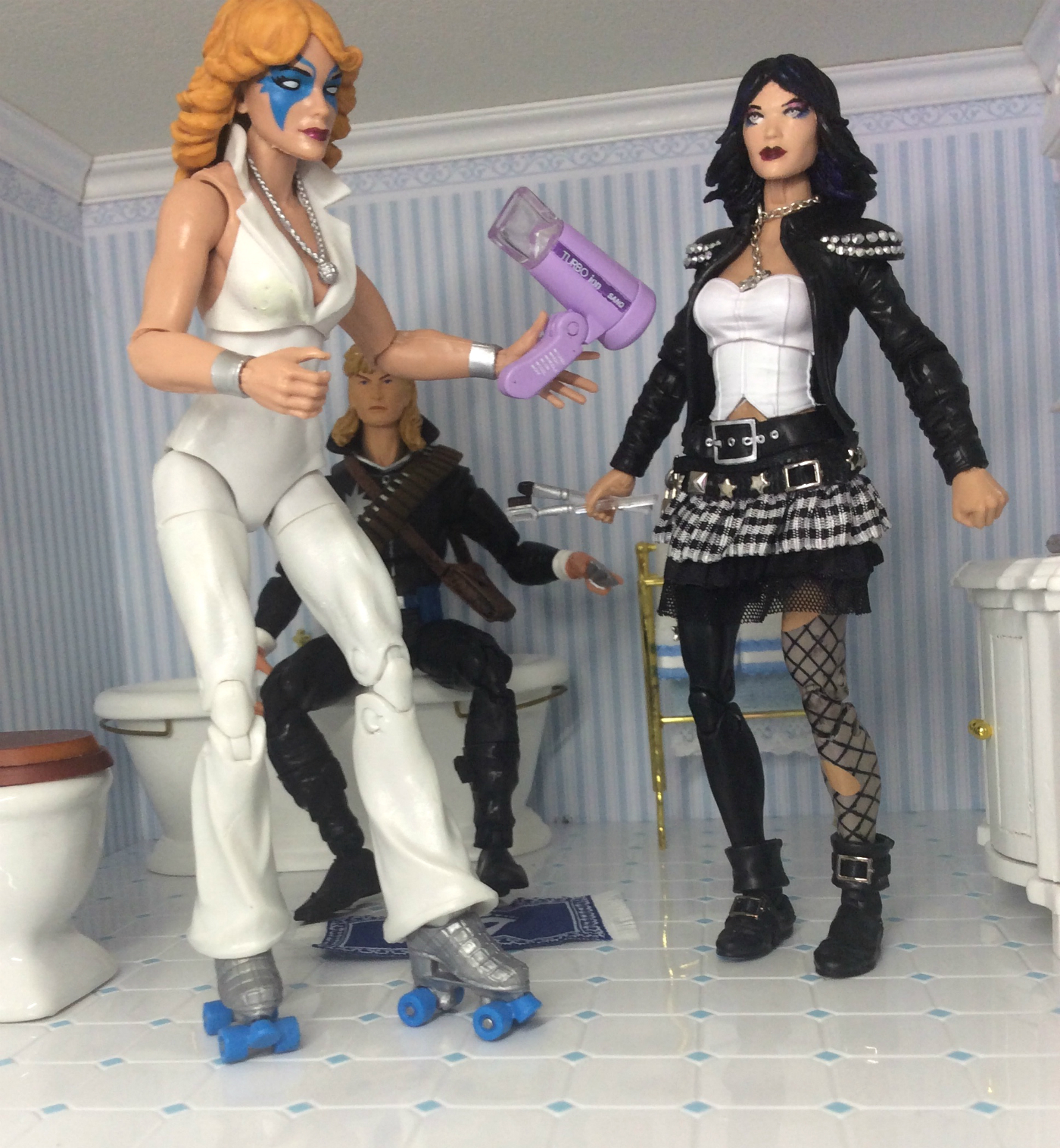In this detailed image of a miniaturized bathroom setting, there are three action figures each with distinct appearances. The bathroom features white square tiles with blue diamonds interspersed, blue and white pinstripe wallpaper, and white crown molding. At the back, a male figurine with a mullet hairstyle sits on the edge of a bathtub. He is clad in all black, with leather straps and a purse crossing his chest.

To the right of him, a goth-styled woman is the centerpiece, flaunting a black leather jacket adorned with star studs on her shoulders. She wears a black and white checkered skirt, a white corset, two belts, and fishnets on one leg and stockings on the other. Her black boots are accentuated with buckles, and her bold, dark makeup is complete with black lipstick, eye shadow, and a short hairstyle to her shoulders.

On the left, another woman exhibits a more flamboyant look. She has heavy blue eye makeup that mirrors a koala-like pattern, flowing blonde to red hair, and roller skates with blue wheels. She dons a sleeveless white tank top, white pants, and silver bracelets, while a pearl necklace featuring a spherical pendant hangs around her neck. In her left hand, she holds a purple hairdryer.

The bathroom also contains a toilet beside the bathtub and a gold stand towards the right, partially cut off by the image's border. This meticulously arranged scene portrays a blend of punk, gothic, and retro aesthetics through its detailed figurines and miniature bathroom decor.